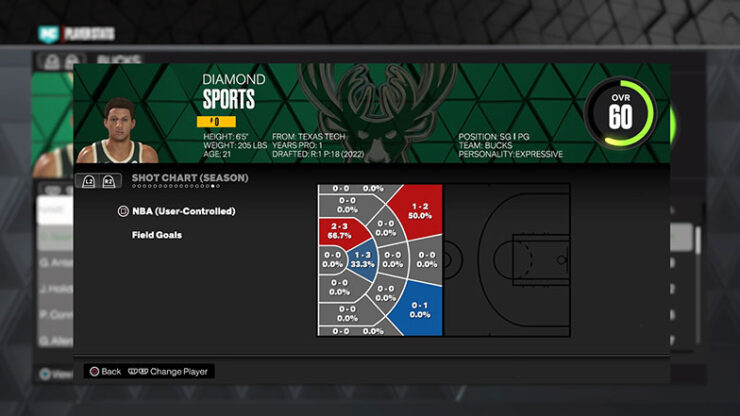The screenshot captures a webpage related to sports, possibly a sports betting or statistics site, featuring a significant pop-up dominating approximately 80% of the screen. In the background, blurry text and imagery are faintly visible. The pop-up in focus displays the title "Diamond Sports #9," which is somewhat difficult to discern clearly. It highlights a basketball player, presumably from the Milwaukee Bucks, depicted with either black skin or very tan white skin. The content appears to showcase the player's season shot chart, illustrating various shot locations with associated numbers and percentages, likely indicating the player's shooting accuracy from different areas on the court.